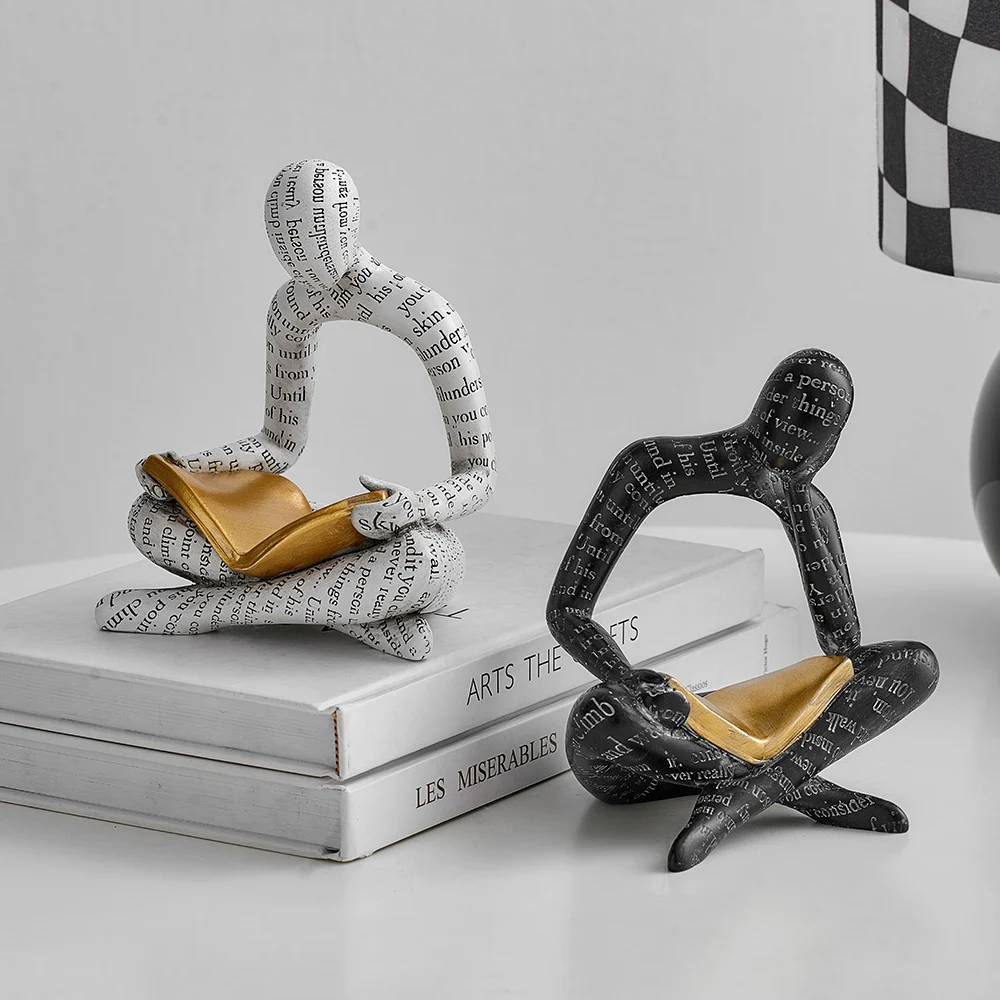The photograph is a contemporary and detailed depiction featuring two sculptural figures in a seated, cross-legged position, reminiscent of the Indian-style pose. These statues are uniquely crafted with only their limbs and heads visible, as their torsos are conspicuously absent. One figure is black and the other is white, and both are adorned with a variety of words inscribed across their forms.

The black figure is positioned next to a stack of books, while the white figure sits atop two white books. The titles of these books include "Les Miserables" and another book possibly named "The Art of Crafts" or "Arts the Something". Each figure holds a solid, bold book in their lap, with one resting its head in its hand and the other reading attentively. The scene is set against a white background, with a black checkered lamp visible in the background, and the figures rest on a black surface, adding to the monochromatic and abstract nature of the photograph.